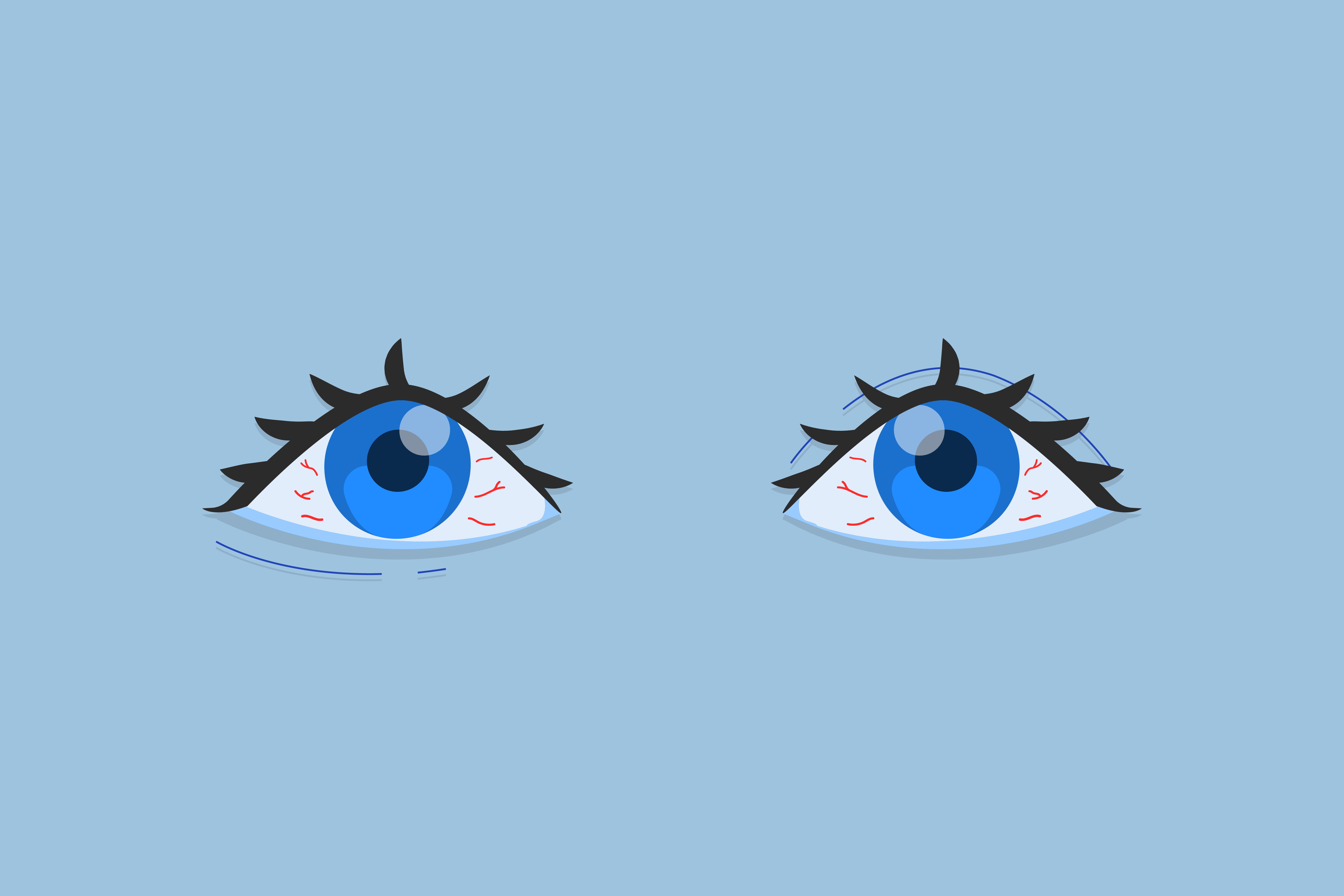The image presents a light blue rectangular background with a pair of striking eyes positioned at its center. These eyes are characterized by their intense blue irises and black pupils. Bloodshot veins are depicted by red lines threading through the whites of the eyes, suggesting a sense of fatigue. Both eyes are accentuated with pronounced black eyelashes. Below the left eye, there is a partially fragmented blue line, while above the right eye, a curved blue line arches gracefully. The light blue background contrasts subtly with the darker blue of the eyes, enhancing their vivid presence. Shadows beneath the eyes add a touch of depth and realism to the composition.